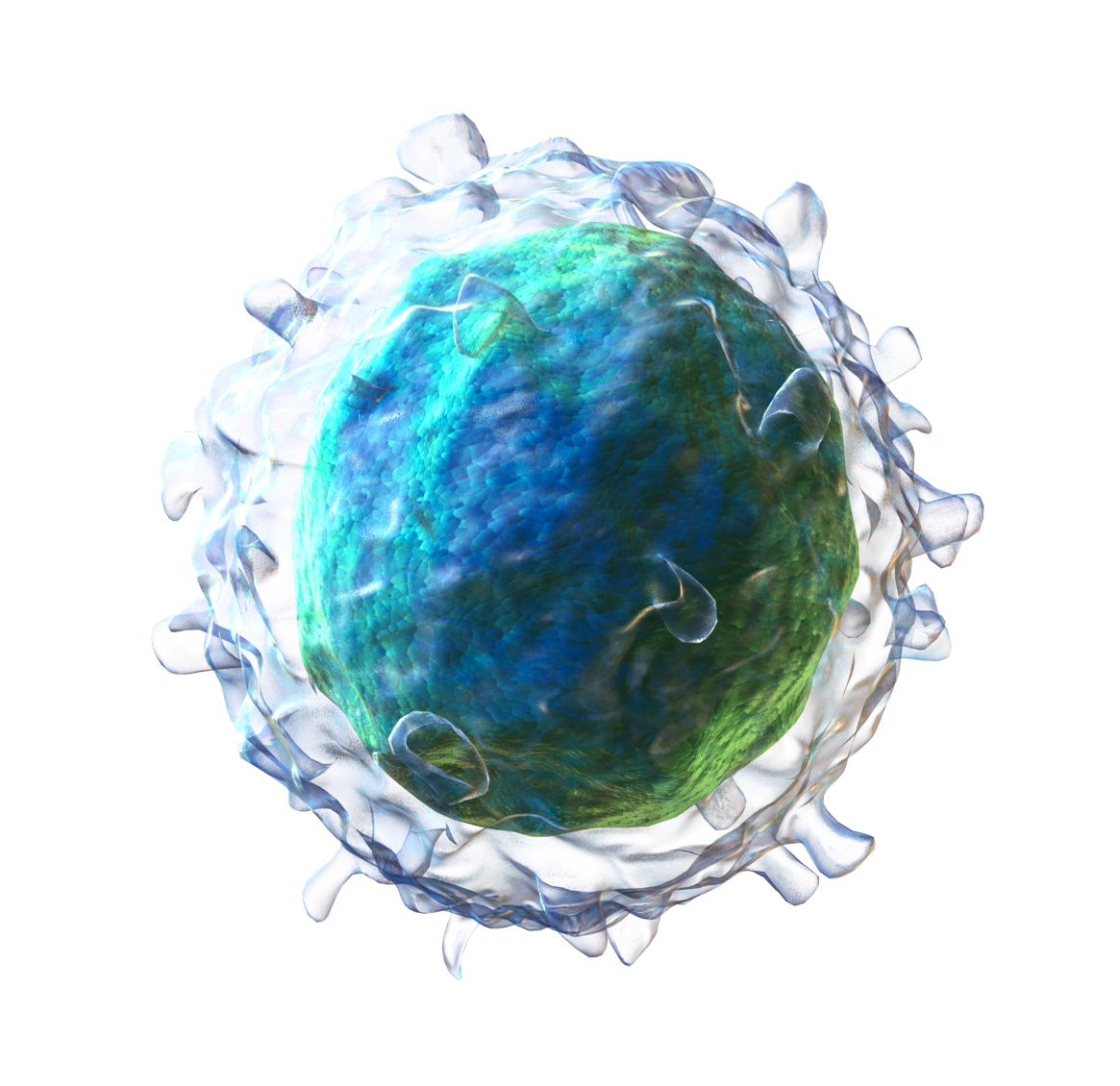The image depicts a circular, possibly digital representation of a microscopic object resembling a germ or cell. At its core is a textured, irregularly shaped globe with a mixture of blues, greens, and occasionally purples, giving it a rock-like but unusual appearance for a rock. Surrounding this central sphere is a clear, bumpy coating that extends outward and gives it a semi-gelatinous look. This outer layer features various jutting elements that resemble tendrils or appendages. The entire structure is encapsulated in a diaphanous, flowing aura with hints of purples, blues, and some areas presenting an aqua hue. The background of the image is stark white, and there are no writings or additional marks. The combination of colors—mainly greens, blues, purples, and some grays—lends a scientific, almost otherworldly aesthetic to the image.